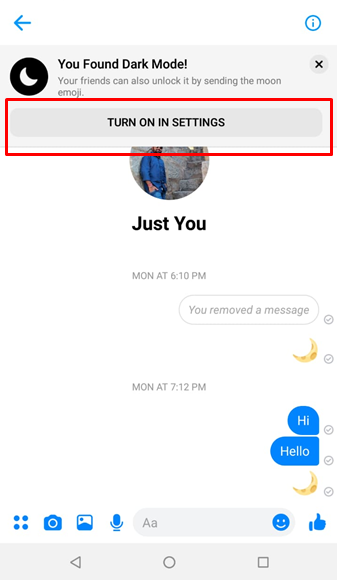This screenshot captures a messaging app interface set against a clean, white background. In the upper-left corner, a blue, left-pointing arrow provides a navigation option. On the opposite side, in the upper-right corner, an information icon represented by an eye enclosed in a circle is displayed.

Centered below the top navigation, a gray notification box excitedly announces, "You found dark mode!" with a corresponding dark mode symbol to its left. Directly beneath this notification, it advises, "Your friends can also unlock it by sending them the moon emoji." 

Underneath the advisory message, a prominent bar labeled "Turn on settings" is emphasized with a red rectangle drawn around it, highlighting it as the key action point.

Further down the screen, a partial picture of a person is visible from their knee to approximately half of their face, making the identity ambiguous. Below this image, the phrase "Just you" is displayed, followed by a chronological exchange of messages.

The conversation begins on Monday at 6:10 PM with an activity notification: "You removed a message," accompanied by a small dark mode moon icon. Following at 7:12 PM on the same day, the messages read, "Hi," "hello," and another dark mode moon emoji. 

At the bottom of the interface, various options for user interaction are available, including icons for uploading a photo, taking a photo, recording audio, sending an emoji, among other functions, providing comprehensive interactive functionality within the app.